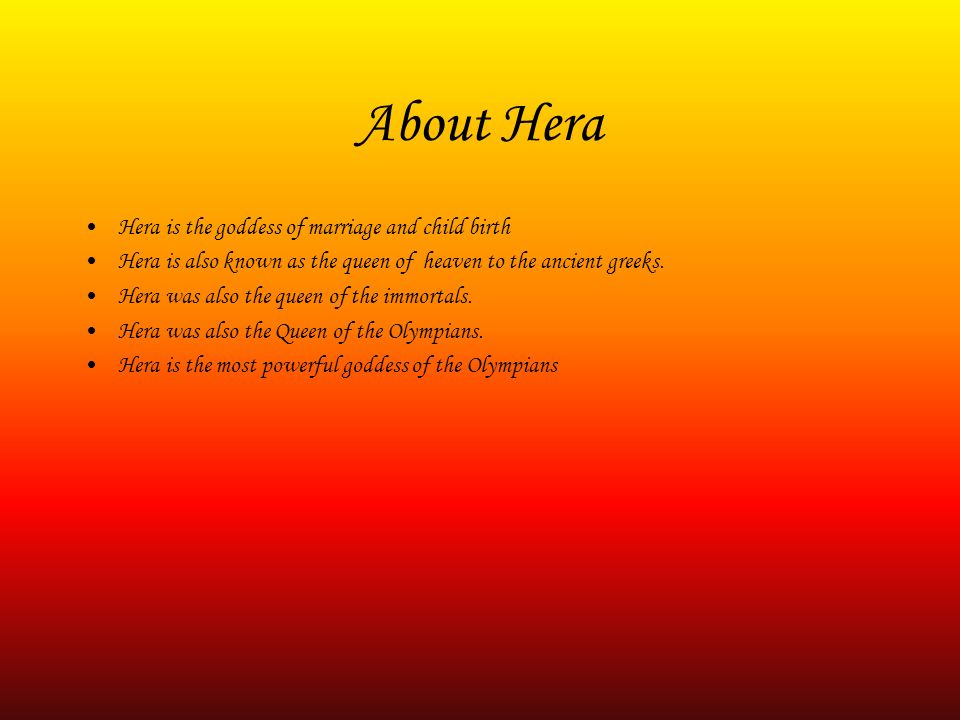The image is a vividly designed card featuring a gradient background that transitions from bright yellow at the top to a deep crimson red at the bottom. The central focus is the text, which is headed by "About Hera" in large, bold font. Below the heading, a series of bullet points provides detailed information about Hera, emphasizing her importance in ancient Greek mythology. The first bullet point identifies Hera as the goddess of marriage and childbirth. The second point states that she is also known as the Queen of Heaven to the ancient Greeks. The third bullet marks her as the Queen of the Immortals, followed by another noting her title as the Queen of the Olympians. The final bullet point highlights Hera as the most powerful goddess among the Olympians. The text is styled with a slight flourish, enhancing the elegant presentation of the information.